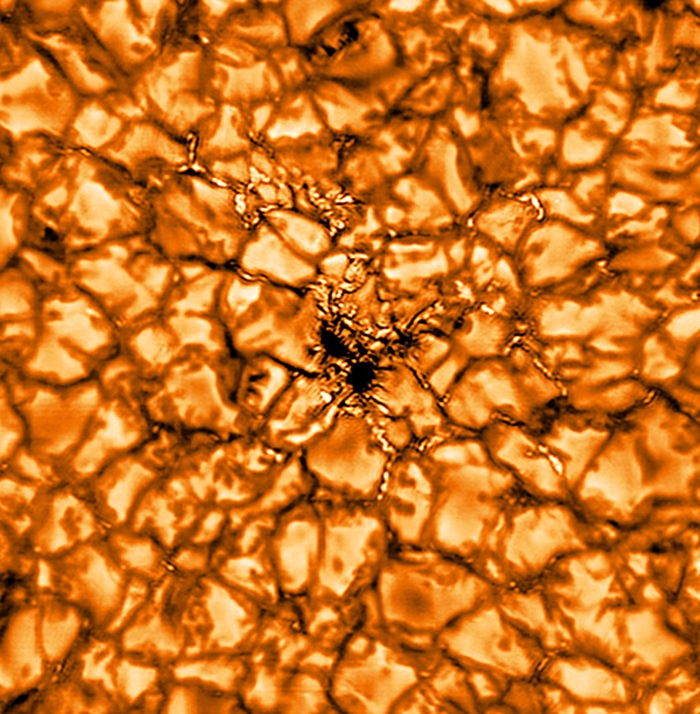The image is a detailed digital scan that resembles a microscopic view, potentially of cells or germs, featuring a vivid color palette of primarily gold and orange hues against a black background. The central focus of the image includes two prominent black empty spaces resembling cracks in glass, bordered by smooth-textured, gold-colored rock-like objects clustered together. The intricate design gives the impression of a modern, abstract wallpaper. The overall composition highlights the contrasting interplay between the bright rock-like formations and the dark, fragmented voids.